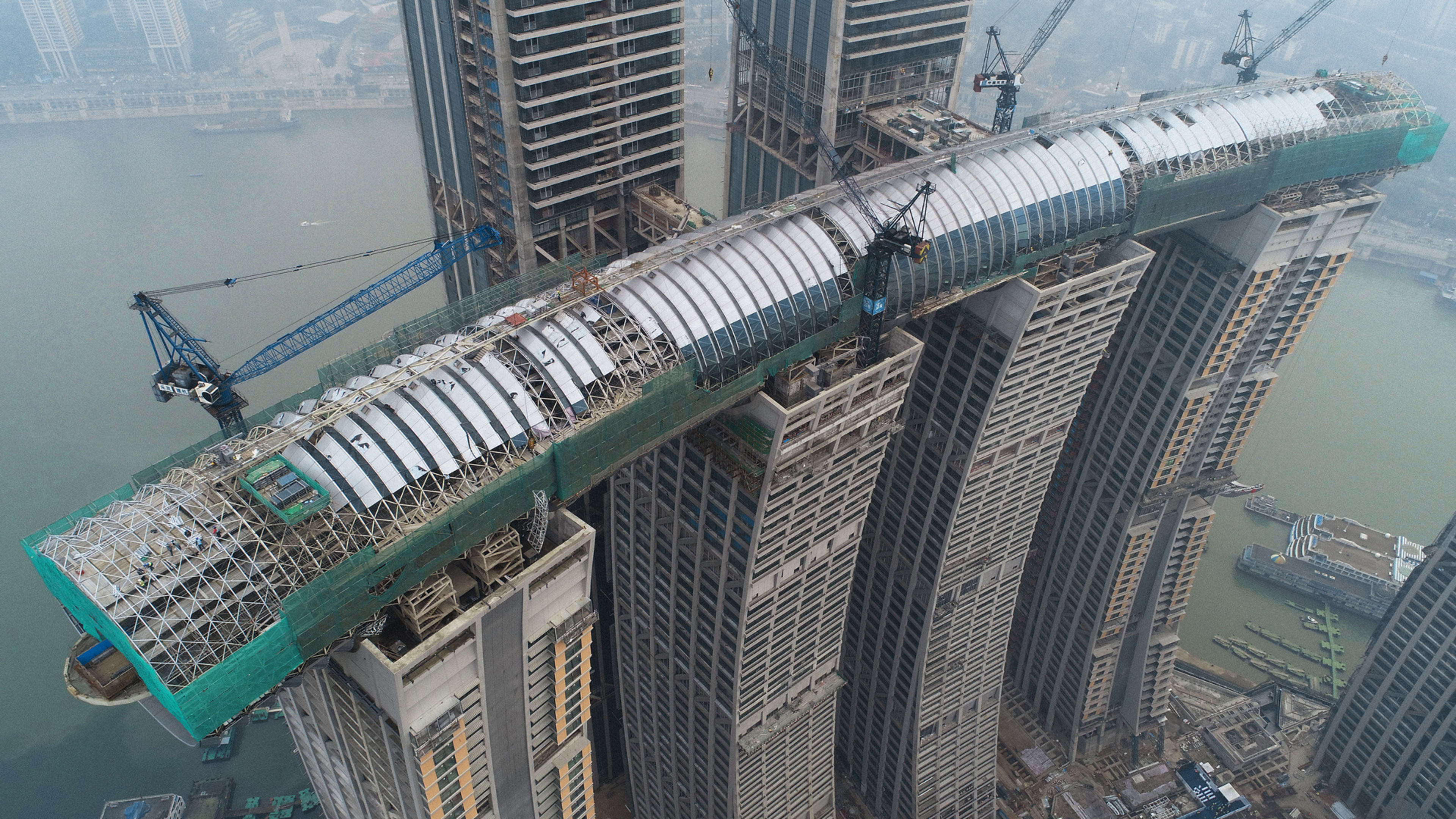The image, captured from an aerial perspective likely using a drone, depicts a bustling daytime cityscape shrouded in a light fog or smog. At the forefront, four intricate and curvy skyscrapers dominate the scene, with ongoing construction atop them involving a connecting structure composed of white panels and green elements, potentially resembling a greenhouse or an overhead walkway. Numerous cranes, both on the left and right sides of the skyscrapers and atop them, indicate active construction, surrounded by the efforts of engineers and workers. The background reveals a water body, possibly a river, with ships, boats, and piers visible. Across this river, additional skyscrapers and smaller buildings recede into the hazy distance, completing the urban panorama.